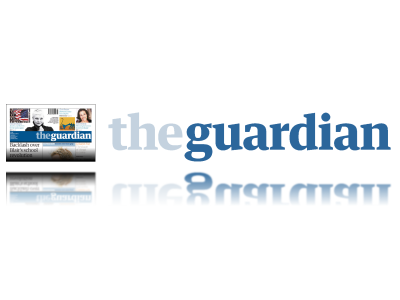This image is a horizontal rectangle, with no distinct borders. On the left, there is a very small horizontal rectangular image with a light gray or black border. This small image appears to be a picture of either a newspaper or a reading material. Central to the image is a medium blue-toned horizontal rectangular section. Just left of its center, 'the Guardian' is written in all lowercase letters. 'The' is in a possibly light blue or white font, while 'Guardian' is bolded in white. 

In the upper left corner of this section, there is an image of the American flag. In the upper right, there is a picture of a woman. Continuing down, beneath 'the Guardian', there appears to be a headline in black font on a white background. This text appears to reflect below. Adjacent to this section, another instance of 'The Guardian' logo is present. Here, 'The' is in light gray, and 'Guardian' is in the same medium-toned blue, all lowercase. This logo also has a mirrored reflection effect below it.